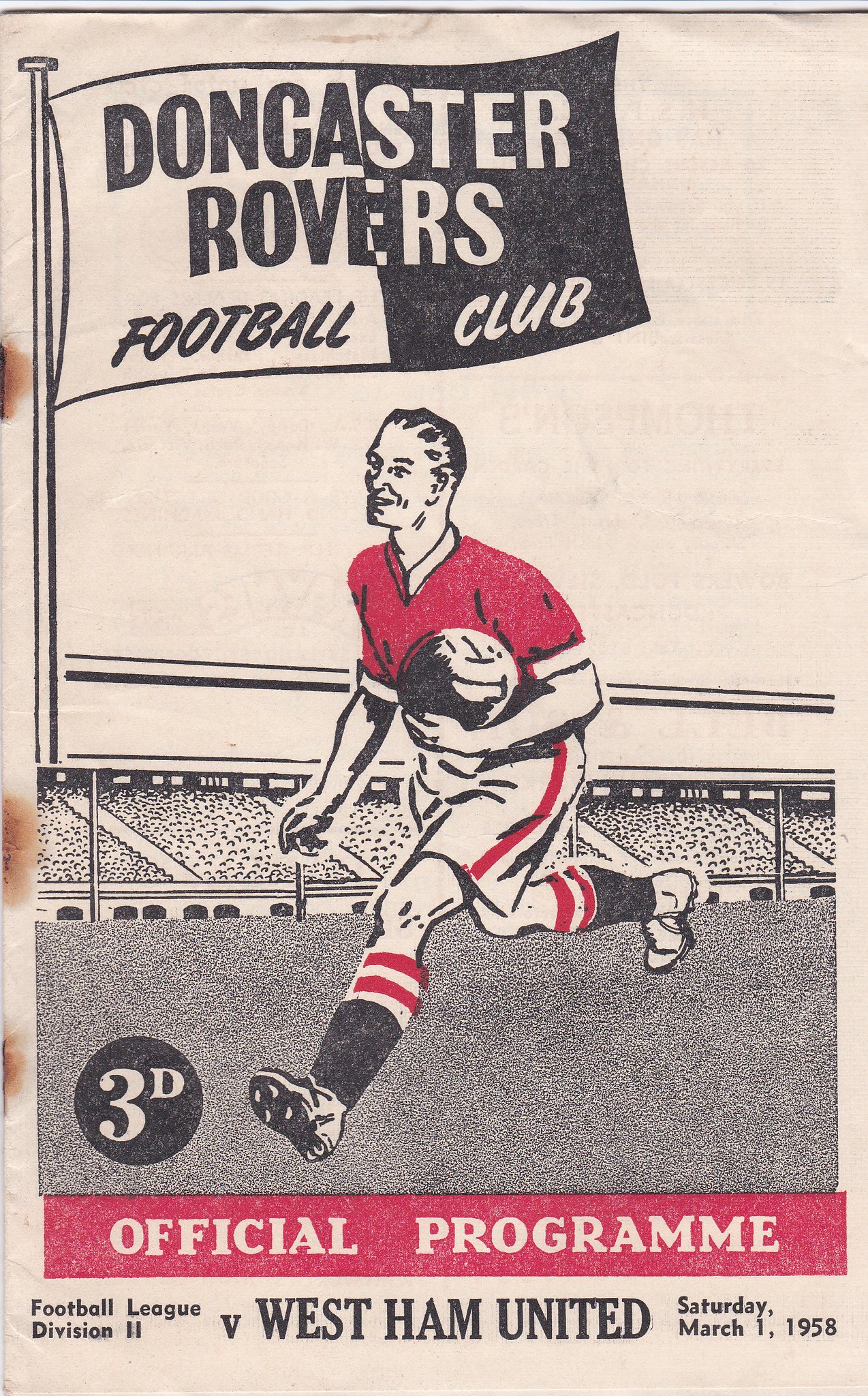This detailed descriptive caption summarizing the three provided captions emphasizes shared and repeated elements:

This image depicts an old-fashioned football program cover from Doncaster Rovers Football Club, dated Saturday, March 1, 1958. At the top left, a flag with a distinctive half-black and half-white design prominently displays "Doncaster Rovers Football Club." Below the flag, a pole extends from the top to the middle of the page. Central to the image is an illustration of a soccer player in a red shirt, white shorts with red stripes, white socks with red stripes at the top, and cleats. The player is shown running to the left with a soccer ball tucked under his right arm, his right leg forward, and his left leg back. The background features bleachers filled with stylized, indistinct spectators. At the bottom, the text reads "Official Programme" in white capital letters on a red background, followed by "Football League Division 2" in black text, and "Versus West Ham United, Saturday, March 1, 1958" spaced across the bottom section. Near the player's foot, there is a black circle with "3D" inscribed within it, indicating the program’s price.